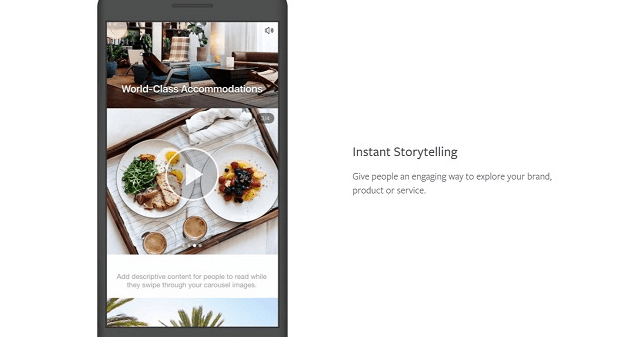The image features a vibrant and engaging promotional carousel designed to highlight different aspects of a brand, product, or service. The scene appears to be set within a cozy, well-decorated living room adorned with a round leather couch, a reclining chair, lamps, curtains, and windows. A smartphone on the left side of the image displays a picture of the living room at the top. 

In the background of the image, there are green palm leaves with a clear blue sky, adding a touch of nature to the setting. A prominent white text overlay reads "World Class Accommodations" and another smaller text "3-4". Toward the left of the image, there’s a spread of food items, including bread, greens, eggs, and yolks, with text that says "Sheet of White." Two drinks are positioned at the bottom of this section. On the right side, a mix of berries and two neatly folded towels at the top right add to the sense of comfort and hospitality.

The bottom of the image suggests adding descriptive content to the carousel, inviting viewers to engage by swiping through. Unfortunately, the overall imagery and text quality appear grainy and low-resolution, detracting from the otherwise inviting presentation.